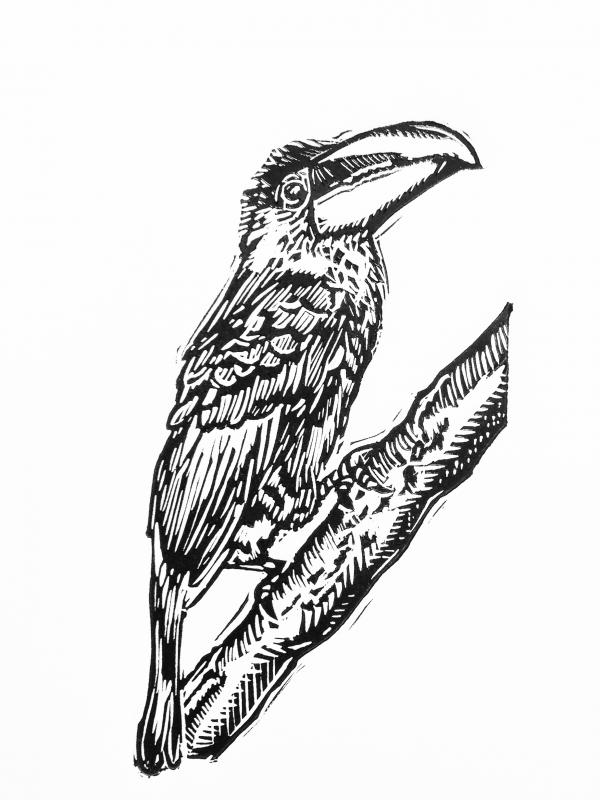This image features an artistic representation of a toucan, depicted in a detailed black-and-white scratchboard style. The artwork portrays the toucan from its right side, perched on a branch that extends from the bottom left to the mid-right of the image. The background is a simple white, suggesting it might be either on a PNG with a white or translucent background or perhaps just white paper. The toucan's large beak is prominently shown, curving over the bottom portion, and the bird is angled upward. It displays a mix of finely detailed small feathering along the top of its head and back, and the longer strokes define its tail feathers which end in a slightly loopy shape. The bird's talons are gripping the branch firmly. The overall dimensions of the image are approximately 2 inches across by 4 to 5 inches long. There is no text, other objects, or visible artist's signature present in the image.